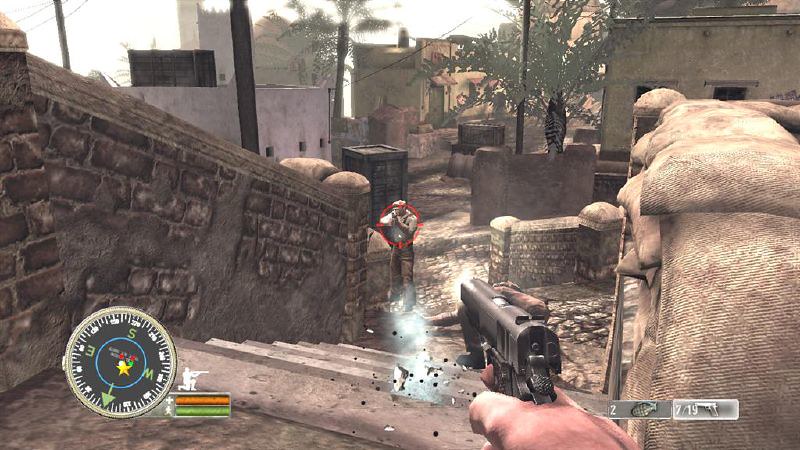The image appears to be a screenshot from a video game, depicting an intense action sequence. In the foreground, the close-up of a man's hand gripping a gun suggests he is about to shoot. He stands on a staircase, and an imposing lion statue can be seen to his right. At the bottom of the staircase stands another man, also holding a gun, with a red circle highlighting him. Evidence of a recent shot is visible, as a bullet appears to have struck the stairs. Overlay graphics include a compass and status bars in orange and green, showing character health or status. The background features detailed environment elements: a sidewalk, additional buildings, a gray sky, and some trees, enhancing the sense of immersion in this virtual world.